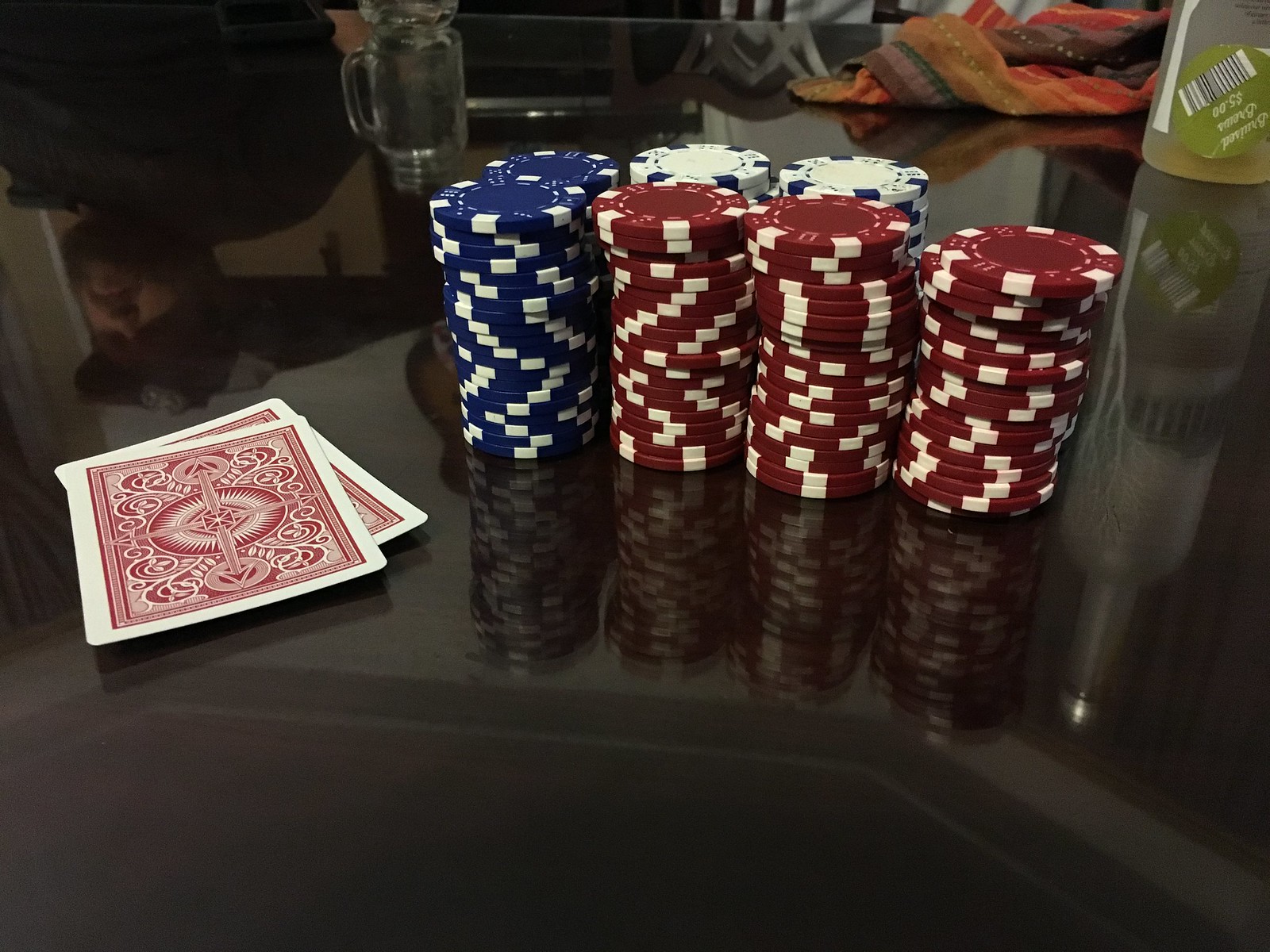This horizontally oriented photograph captures a black table set up for a game. Positioned on the left middle part of the table are two playing cards lying face down, featuring a white border and a red design. Next to the cards, seven neatly arranged stacks of poker chips are visible: two blue stacks, two white stacks, and three red stacks.

In the backdrop, the reflection of a man in a black shirt and black hat is discernible in the upper left corner. He also has a glass mug beside him. On the right-hand side of the table's reflection, a bottle is noticeable. Behind this bottle, a piece of multicolored cloth in hues of red, orange, green, brown, and gray adds a touch of vibrancy to the scene.